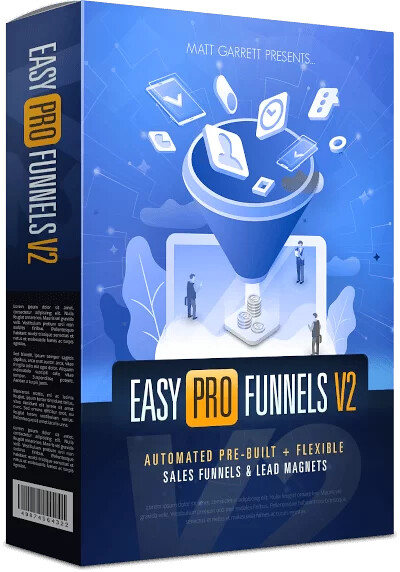The image depicts an angled, rectangular portrait-shaped box that stands on its end against a white background. The box, which is reminiscent in shape of a bundle or ream of office paper, is predominantly blue with a gradient from darker blue at the bottom to a lighter medium blue towards the top. The front of the box features the title "Easy Pro Funnels V2" prominently in the lower half, with the subtitle "Automated Prebuilt + Flexible Sales Funnels & Lead Magnets" written beneath it in smaller font. Above these words, there's an illustration of a blue funnel into which various digital objects such as cell phones, clocks, and contact information tiles are being tossed. At the mouth of the funnel are three small office workers in professional attire and a pile of stacked coins at the funnel's base. The top of the front side reads "Matt Garrett Presents." The left side of the box, which is visible due to the angled presentation, repeats the title "Easy Pro Funnels V2" rotated 270 degrees along with a UPC symbol at the bottom.